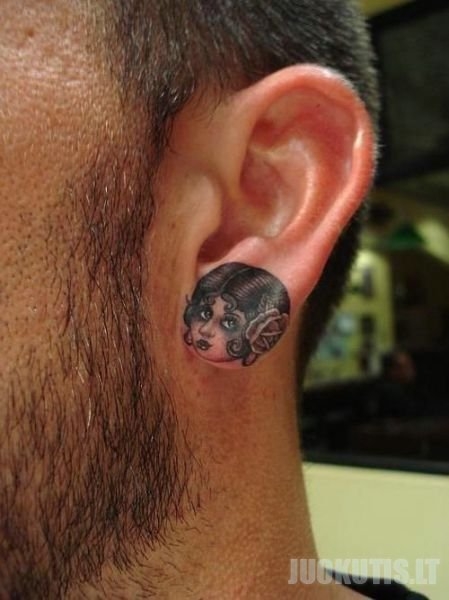The photograph captures the left side of a man's face, focusing prominently on his ear and an intricate tattoo on the earlobe. The tattoo features the face of a woman with short, curled hair down to her chin, adorned with a flower, which appears to be a rose, in her hair. She has a rounded face, big round eyes, a defined nose, and red pouty lips. The man has a brown, thin beard with a few gray strands, and his short brown hair is visible above his ear. In the lower right corner, the text "JUOKUTIS.IT" is printed in faded white letters. The background on the right side is blurry and indistinct, possibly depicting a wall with a window, suggesting an indoor setting. Colors in the image include brown, gray, tan, black, red, green, and yellow. The primary focus remains on the detailed tattoo and the man's ear, symbolizing a recent visit to a tattoo parlor.